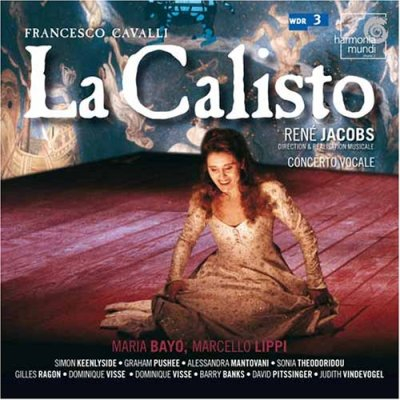This detailed image depicts what appears to be a CD or vinyl album cover for Francesco Cavalli's "La Calisto." Prominently at the top, large white text spells out "La Calisto," and "Francesco Cavalli" is also inscribed. Central to the cover, a woman is kneeling on a broad, red, wooden floor composed of several red boards. She is wearing an elegant, tan floral dress adorned with various unrecognizable dots and images, holding her dress and smiling warmly at the camera. The background features a wall heavily decorated with superimposed photos and artwork, adding depth to the visual composition. Above, "Harmonia Mundi" and "WDR3" are marked clearly. The lighting highlights her face beautifully, indicating a professional and well-lit photography setup. The album credits name Rene Jacobs prominently at the top right and include numerous names at the bottom: Marie Belli, Marcello Lippi, Maria Bayo, Simon Keenlyside, Graham Pushee, Alessandra Donovany, Judith Malafronte, David Pitt, Barry Banks, and Dominique Visse. This intricate and elegant cover encapsulates a high-quality classical vocal or opera collection directed by Rene Jacobs with performances by various artists.